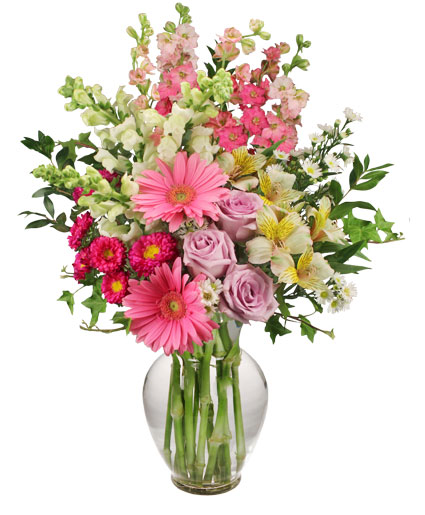This image displays a beautifully arranged bouquet of flowers in a clear, heart-shaped glass vase with a subtle, thinner neck and wider bottom. The transparency of the vase allows a clear view of the green stems immersed in water. The bouquet fans out into a diamond shape, with taller blooms at the top and wider elements on the sides, creating a balanced, eye-catching display. The flowers appear very fresh, almost pristine, hinting they could be artificial. The arrangement features a rich variety of colors and types: two medium pink daisies in the front, three light pink roses, several dark pink flowers with bright yellow centers, and flowers with pale yellow petals and darker yellow centers. Adding to the diversity, there are tall stems with buds and blossoms in shades of white, light pink, and medium pink. The striking white background suggests this image might be from an online florist's catalog, emphasizing the bouquet's multicolored, vibrant appeal.